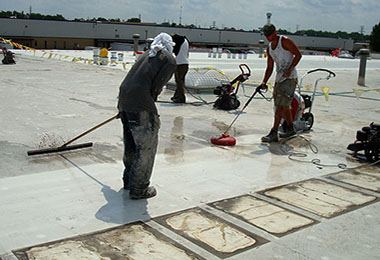The photograph captures an outdoor scene of a man-made area, likely a parking lot, where multiple workers are engaged in cleaning or possibly flattening cement. The ground is a combination of white and gray hues. On the left side of the image, one worker, dressed in a tank top, shorts, and boots, is using a wiper to clean dark, dirty water off the surface. To his right, another worker, clothed in a long-sleeved shirt, pants, and boots, is operating a machine on the ground. In total, there appear to be three or four men in the picture, some holding tools, and one individual standing with his back turned to the camera. The bright sun reflects off the man in the tank top, indicating a hot, sunny day. In the distant background, a wide, white building is visible against a blue sky dotted with white clouds. The color palette includes gray, tan, white, black, yellow, orange, and red.